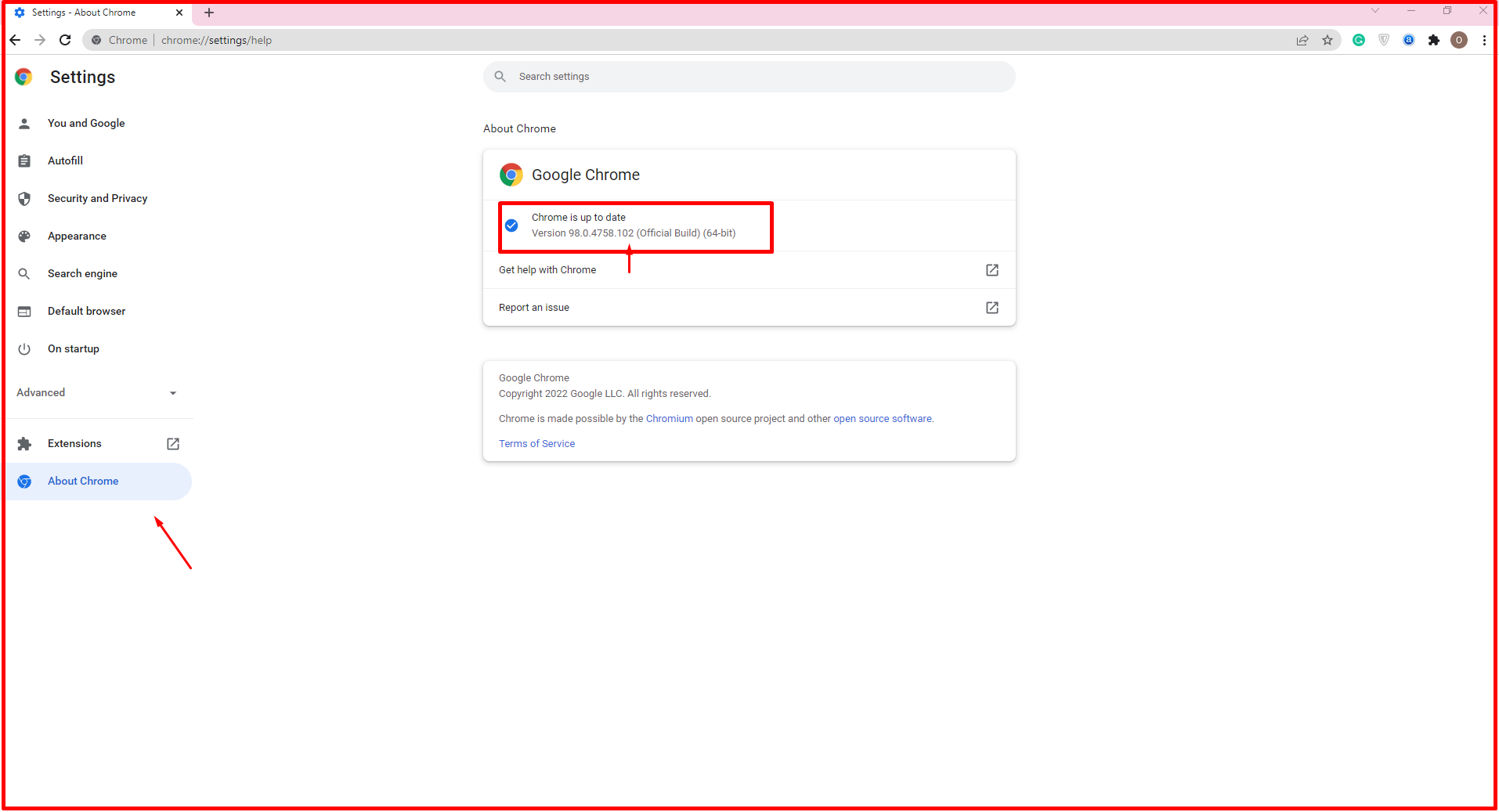The image depicts a chrome settings page. The background is predominantly white and outlined in red. At the top, a pale pink banner stretches across the screen. In the top left corner, "Settings" and "About Chrome" are written in white against the pink background, using a black font. Adjacent to these, a blue gear icon representing the Settings. Directly below this area are navigation arrows: a black arrow pointing left and a grayed-out arrow pointing right, followed by a black Refresh or Reload button. To the right, there is a gray search bar with the text "Chrome" inside it, alongside "Chrome Settings Help".

Beneath the search bar, the page prominently displays the Chrome icon with the word "Settings". Below this header, a series of options are listed in black font:
1. "You and Google" accompanied by a small person icon.
2. "Autofill".
3. "Security and Privacy".
4. "Appearance".
5. "Search Engine".
6. "Default Browser".
7. "On Startup".

Additionally, at the very bottom in gray font, the word "Advanced" appears, followed by a black puzzle piece icon with the label "Extensions".